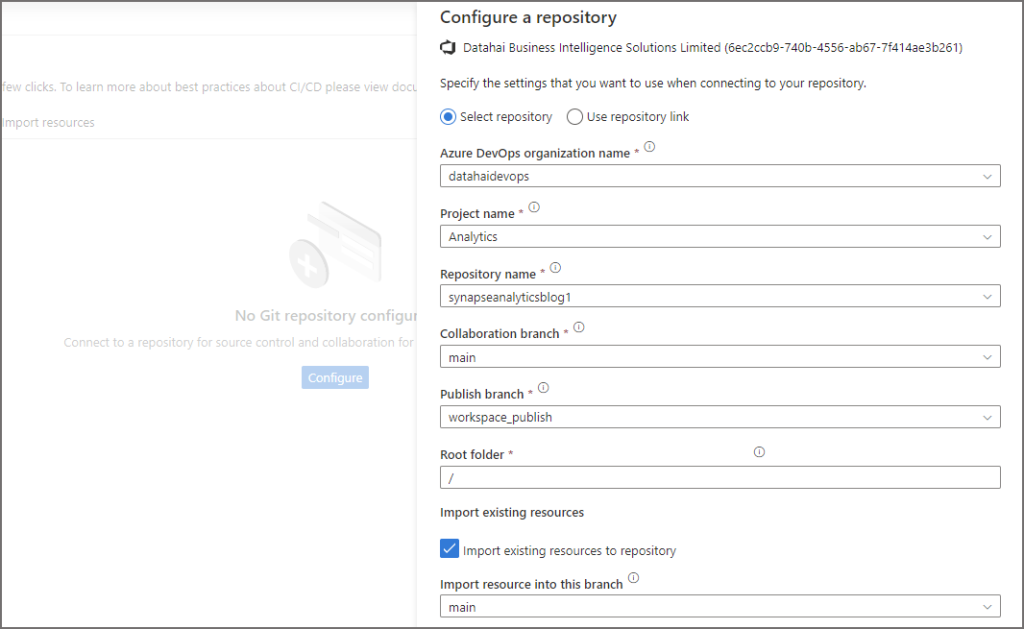This detailed image, captured from a computer screen, depicts a process for configuring a Git repository. On the left-hand side, partially obscured gray text over a white background states: "No Git repository configured. Connect to a repository for source control and collaboration." Interrupting this text is a prominent blue "Configure" button. 

At the top of the image, the title "Configure a Repository" indicates that the user likely clicked the blue button. Below the title, it displays "Data High Business Intelligence Solutions Limited" followed by a lengthy alphanumeric string. A prompt instructs the user to "Specify the settings that you want to use when connecting to your repository". 

The user has selected "Select repository" rather than "Use repository link". Further down, fields are visible for entering an "Azure DevOps organization name", where "data high DevOps" has been typed. A blue check mark is selected next to an option that reads "Import existing resources to repository", suggesting this feature has been enabled.